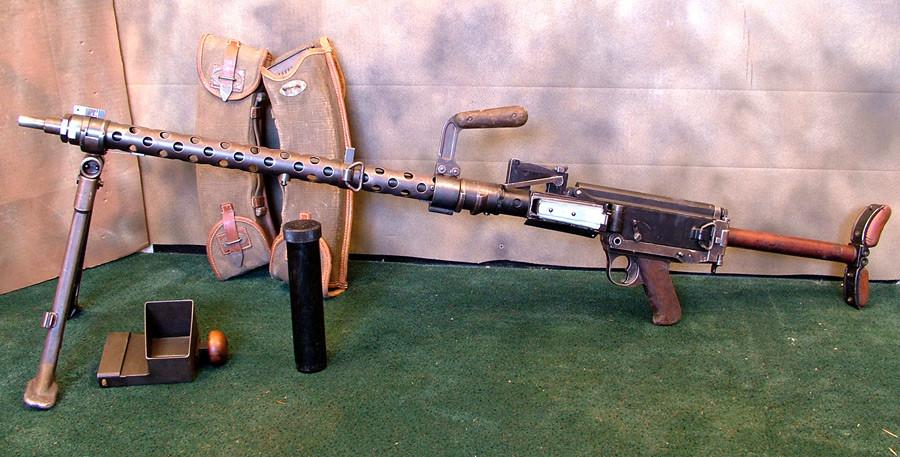The photograph is a horizontally aligned rectangular image, showcasing an imposing machine gun prominently centered on a green, somewhat dirty-looking astroturf surface. The backdrop comprises a rectangular, beige brick wall, casting subtle shadows and lending a textured contrast to the scene. Flanking the gun are two brown leather pouches with buckled closures, leaning against the wall, likely intended for storing gun parts or ammunition magazines.

The machine gun, possibly a .50 caliber due to its size and structure, is positioned on a two-legged stand at its left end where the barrel begins. The barrel is lengthy, silver in color, and characterized by numerous circular vents along its length. Midway up the barrel, a metal turn handle is visible, suggesting it might be used for adjustments. The right side of the gun features a wooden stock and an old-fashioned wooden handle, indicative of a vintage design. The handle section and stock are both grounded on the turf.

In front of the gun and slightly to the left, there's a black cylindrical canister with a silver top, possibly an ammunition container, along with a diminutive metal box adjacent to it. The overall visualization is detailed with elements emphasizing the gun's size, the ammunition containers, and the ambient storage pouches, composing a scene rich in historical and functional aspects.